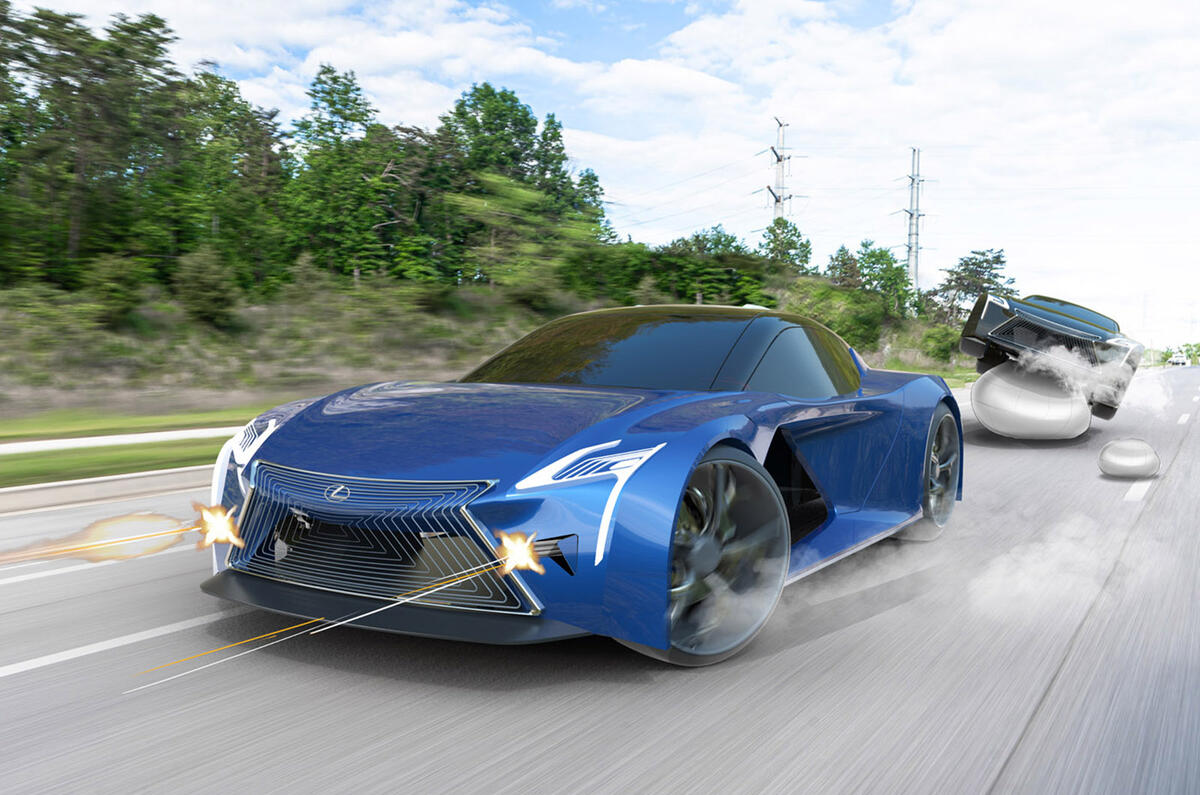This captivating image portrays two high-performance Lexus sports cars zipping down a paved road with a clear blue sky and fluffy white clouds overhead. The focal point is a sleek, modern blue Lexus in the foreground, its heavily tinted black windows and stunning grille accentuating its luxurious appeal. The car's front lights have been creatively edited to appear as if they are emitting dramatic yellow laser-like explosions. The tires exude smoky effects, suggesting immense speed and power. 

Trailing behind it, another edited blue Lexus is seen partially airborne, seemingly navigating over a shiny, metallic rock-like structure with gray bubbles beneath it, contributing to an overall futuristic and animated ambiance. Smoke billows from this second vehicle, adding to the dynamism of the scene. The background reveals green trees, though they appear blurred, indicating the high velocity at which these cars are traveling. The entire composition is infused with energetic and surreal elements, giving it a distinct animation-inspired aesthetic.